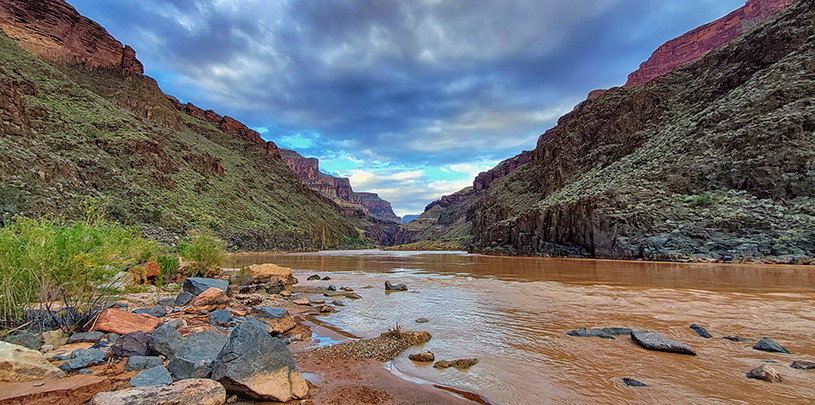The photograph captures a scenic river flowing through a rugged canyon, flanked by mountains on each side, reminiscent of the Grand Canyon. The river, with its rust-colored, muddy water, winds diagonally from right to left in the foreground, revealing multicolored rocks ranging from slate gray to reddish hues along its shoreline. The sandy banks exhibit a similar reddish, rust-colored tint, indicative of sedimentary soil. The canyon's steep, somewhat weathered walls rise up with patches of light green foliage, likely shrubs and low bushes, and are punctuated by rocky outcroppings with shades of brown, gray, and reddish tones.

The upper sections of the canyon walls form a V-shape, with the sky visible in the middle, appearing lower on the right side. The sky is a dynamic mix of blues, grays, and whites, with clouds stretching across the frame, adding a dramatic contrast to the rugged landscape below. The stone walls, rough and bumpy, display signs of erosion, with loose rocks and fine greenery clinging to their surfaces. There's a notable bright red rock or sunlight reflection on the upper right side, contributing to the overall palette.

In the background, the canyon walls seem more vertical, displaying layers of rocks and greenery. The foreground on the left side shows larger, angular gray rocks, possibly recently fallen, with a muddy, silty bank that might contain some clay. Sprouting from the banks are thin-stalked shrubs with light green and yellow foliage. The entire scene, with its earthy colors and varied textures, hints at a southwestern U.S. location, captured in a photograph likely taken within the past 15 years.